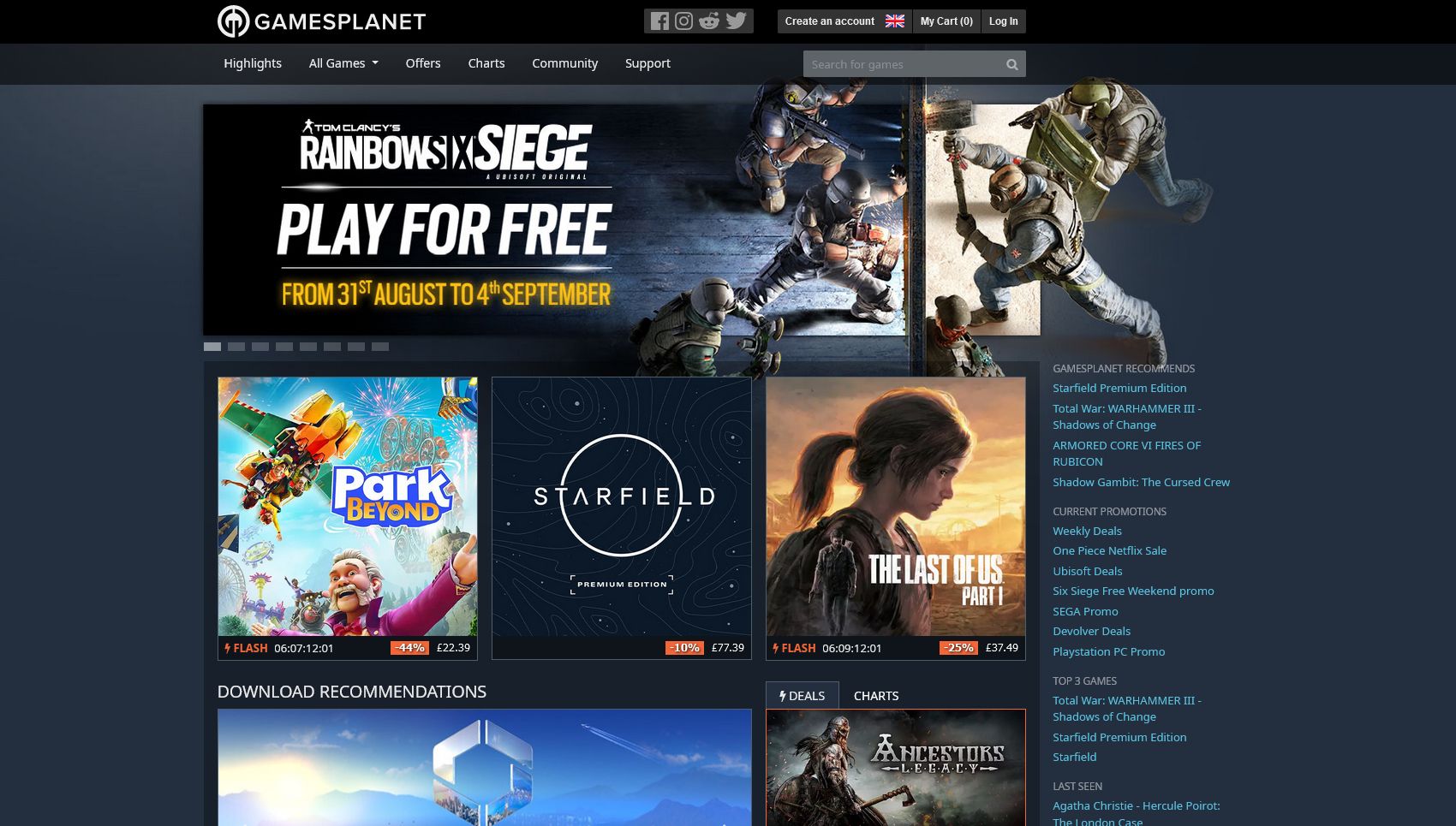The image features a detailed and dynamic homepage for a gaming website named GamePlanet. At the very top, in bold black and white, is the GamePlanet logo. Below this, a sleek gray navigation bar houses icons for Facebook, Instagram, Reddit, and Twitter. The bar includes buttons labeled “Create Emails” in white text, a British flag indicating language preference, and options for "My Cart" and "Login." 

On the left-hand side of the page, vertical menus highlighted in white on a dark background list various sections: Highlights, All Games, Offers, Charts, Community, and Support. Below this menu is a gray search box, subtly labeled "Search for Games" in light gray text.

In the main content area, a black section prominently features the game "Rainbow Six Siege," with a yellow banner indicating a free play period from the 31st of August to the 4th of September. The imagery shows opposing teams gearing up for battle.

Beneath are additional game highlights: "Starfield," "The Last of Us Part 1," and a kitty-themed game reminiscent of "Beyond Park." 

On the right-hand side, under the header "GamePlanet Recommended," featured games include "Starfield Premium Edition," "Total War: Warhammer," "Armored Core 5: Fires of Rubicon," and "Shadow Gambit: The Cursed Crew." 

The bottom section of the page is dedicated to ongoing promotions, with labels in various colors denoting deals from Netflix, Ubisoft, Sega, PlayStation, and PC. There are also banners for special promotions such as weekly deals and free weekend promos for "Six Siege."

In a dedicated "Top 3 Games" section, the website highlights "Total War: Warhammer 3," "Shadow's Unchanged," and "Starfield Premium Edition" among its most recommended titles, all separately showcased for optimal visibility.